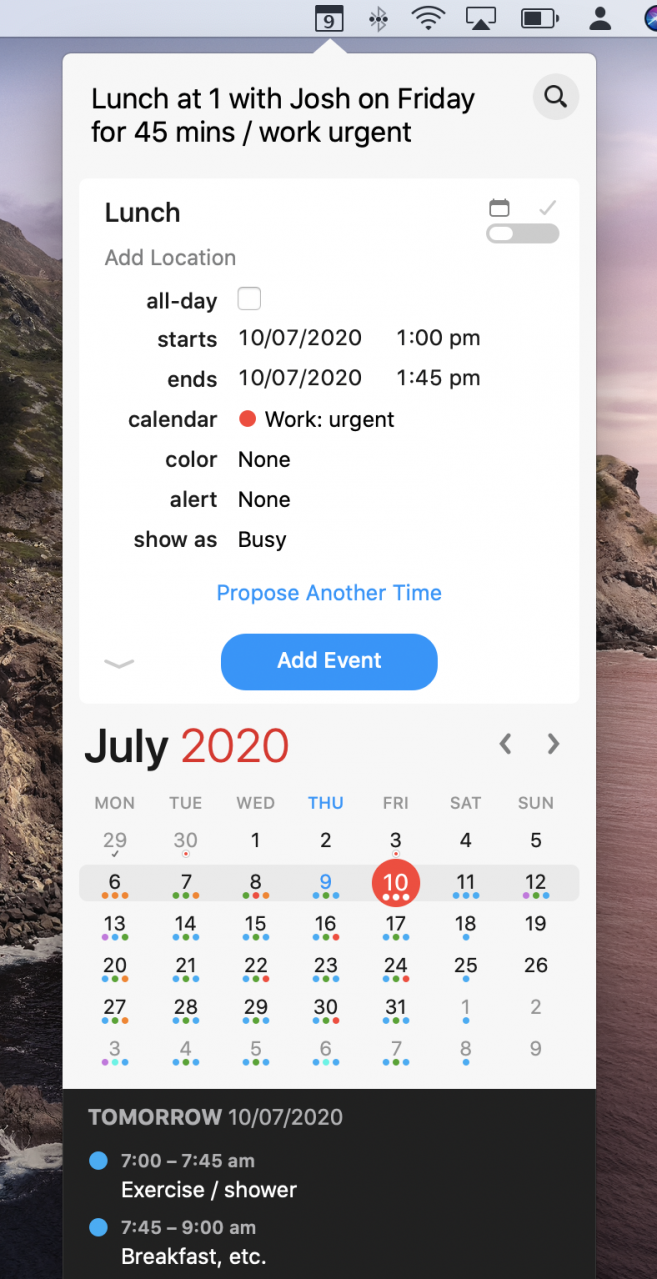The image is a screenshot from a smartphone, displaying the calendar app set against a picturesque beach-themed wallpaper. In the background, there's a scenic view of a beach with rocky formations and towering mountains on the side, all bathed in the warm, serene hues of a sunset sky, tinged with purples and deep mauve.

At the top of the screen, there is a calendar notification represented by a box with the number "9" inside it. The details of the event show "Lunch at 1 with Josh on Friday," scheduled for 45 minutes and marked as urgent work. Below this, more information is listed: "Lunch" with an option to "Add Location", but the "All Day" option remains unchecked.

The event is slated to start on October 7, 2020, at 1:00 PM and end at 1:45 PM on the same day. The event is categorized under a "Work Urgent" calendar, marked with a red dot. Additional details specify that the event's color is set to "None", alerts are turned off, and it is set to show the user as "Busy".

At the bottom of the calendar entry, there are blue links for "Propose Another Time" and "Add Event". The calendar view displayed is of July 2020, highlighting the 10th with a red circle.